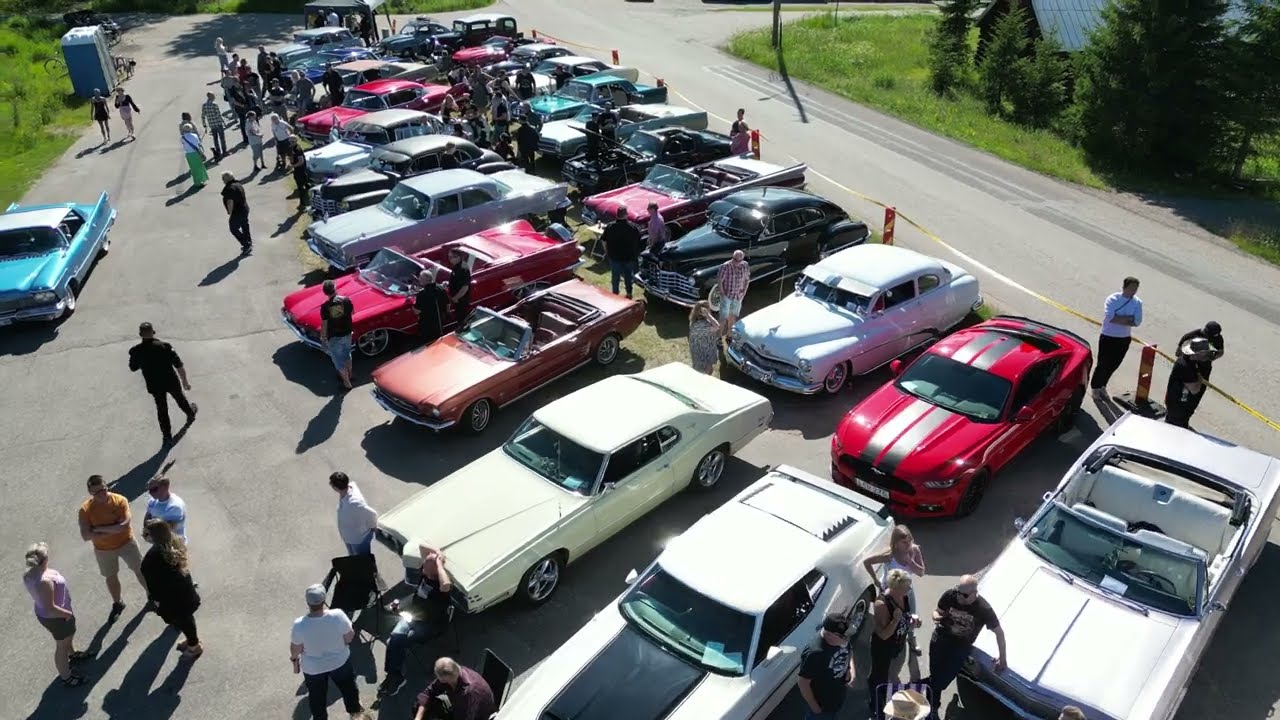The photograph is an aerial shot captured outdoors on a bright, sunny day at an informal car collector’s show. The image showcases a vibrant scene filled with various cars, primarily antique classics and sports cars, all lined up in a diagonal formation across the center from top to bottom. Several convertibles, approximately three or four, are noticeable among the array of vehicles. Surrounding the cars, a crowd of people is seen engaged in conversations and admiring the automobiles. In the background, there are a couple of porta-potties and a building with a tin roof, flanked by pine trees and patches of grass. The scene features a rich palette of colors, including shades of black, white, blue, red, gray, orange, light blue, and green, and no text is visible anywhere in the image. The photograph, possibly taken from a second-story window, encapsulates the lively atmosphere of the midday event.